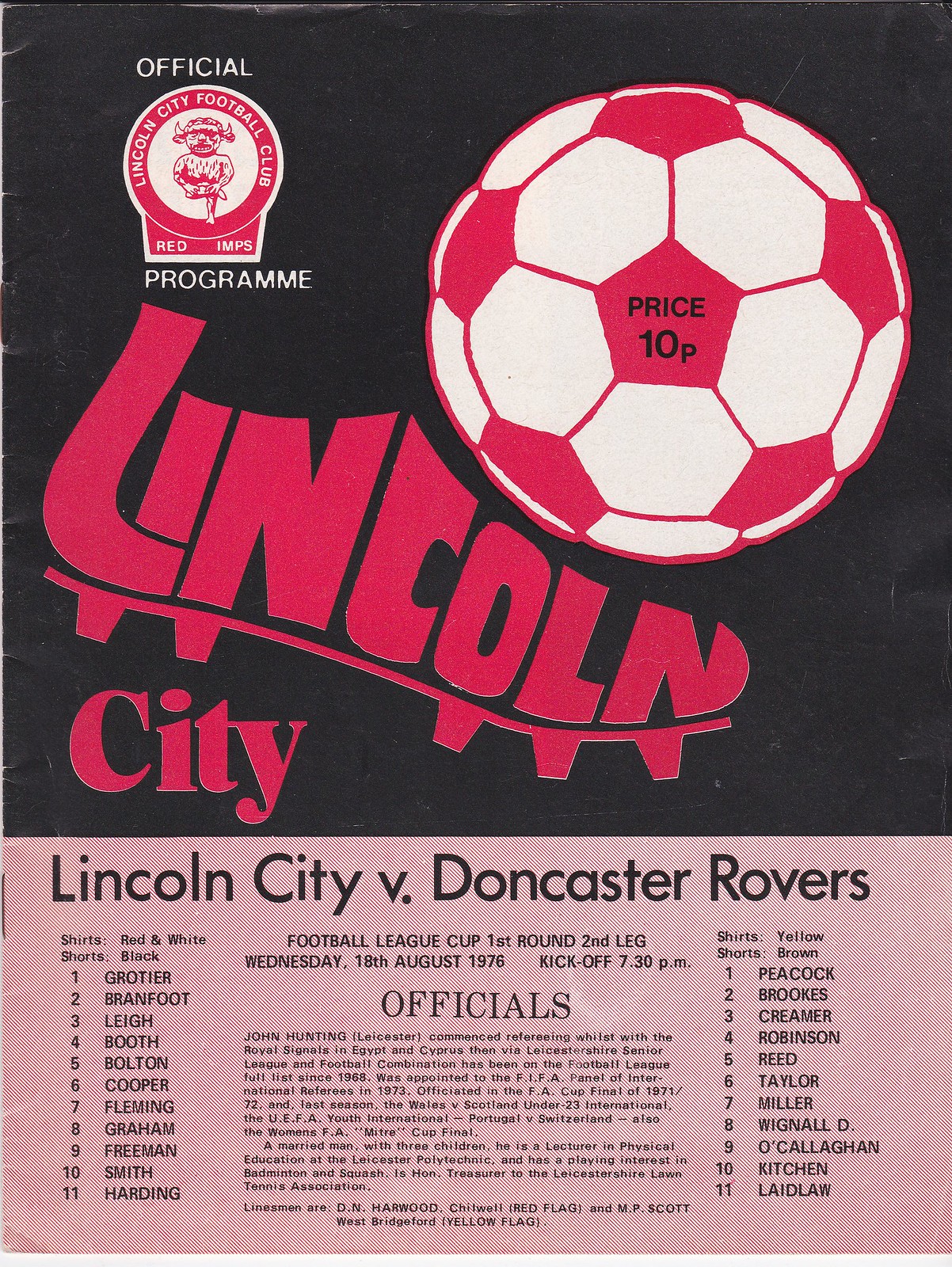The image is the cover of an official program for a football match between Lincoln City and Doncaster Rovers. The cover is divided into two main segments. The top two-thirds of the page feature a black backdrop with a large white and red soccer ball at the center, which has "price 10p" written in black text within a red pentagon shape. Below this, there is an illustration of a foot kicking the ball, where the cleat is creatively drawn using the word "Lincoln" in text form, and the word "City" is in regular red text beneath it. The bottom segment of the cover transitions into a pastel mauve color, displaying "Lincoln City versus Doncaster Rovers" prominently. On the left and right columns, player names and their numbers are listed, distinctively marking the home team's jerseys as red and white with black shorts, and the away team’s jerseys as yellow with brown shorts. The event details are neatly summarized, stating: "Football League Cup, first round, second leg, Wednesday, 18th August 1976, kickoff 7.30pm," followed by the word "officials" and smaller print below it.